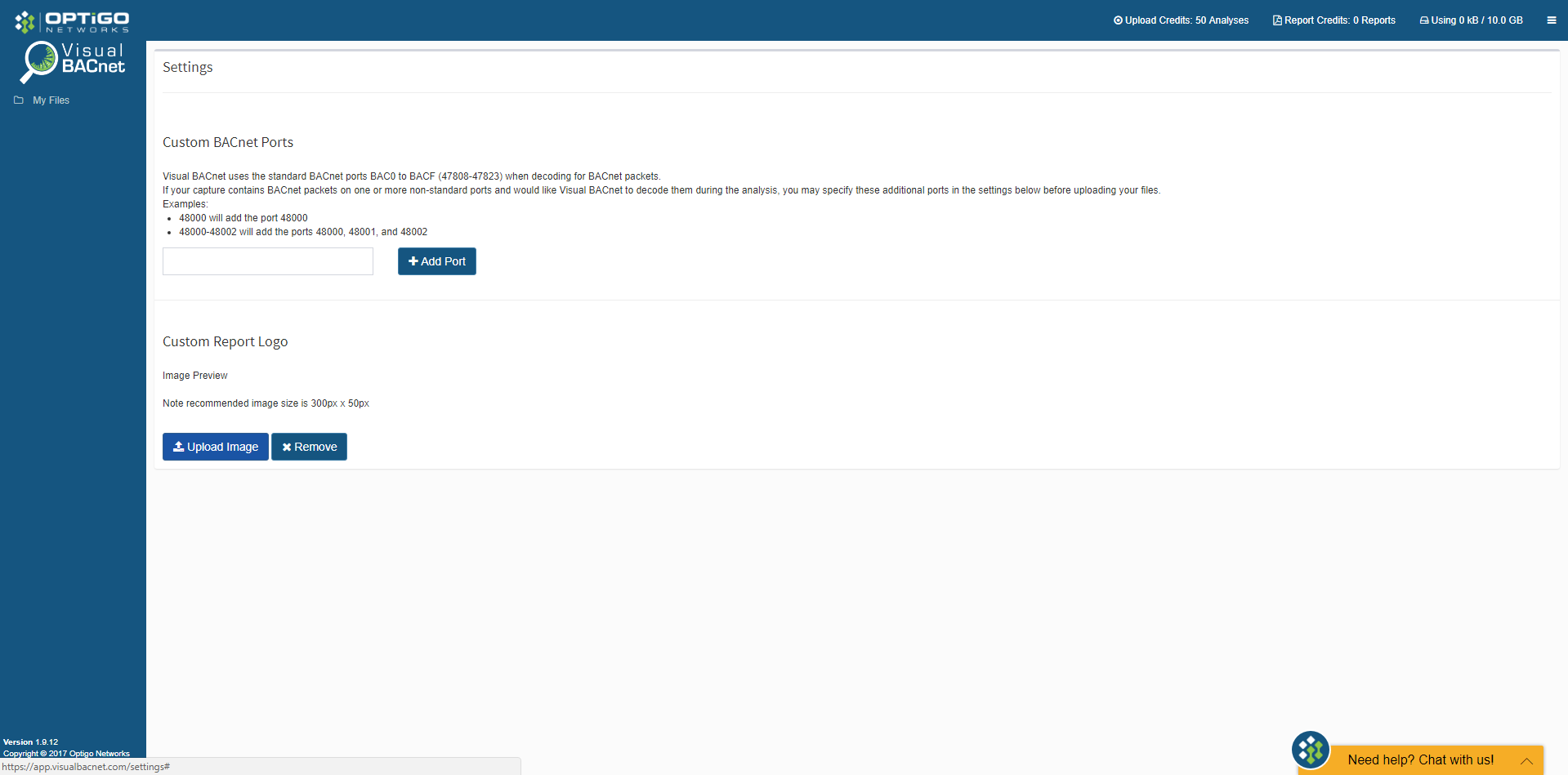This image appears to be a screenshot from a website interface featuring a structured layout with distinct sections and navigational elements. The top section is a blue border, approximately half an inch in height, extending across the top and an inch down the right side. The rest of the background is white.

- In the top left corner within the blue border:
  - There are three white squares: one at the top, two vertically below it.
  - Centered at the bottom middle, there are two white squares with one directly above them. 
  - On the right, there are two white squares.
  
- The blue border contains the bolded white text "OptiGo," and below it in smaller white lettering, the word "Networks."

- Below the text, there is a magnifying glass icon with the handle pointing down to the left:
  - The top left part of the magnifying glass is blue.
  - The bottom right part is green.
  
- To the right of the magnifying glass, the text "visual BACnet" is displayed, with "BACnet" in all capital letters.

- Below this, the words "my files" are present, accompanied by a file icon to its left.

- On the right side within the blue border:
  - There are three white horizontal lines stacked on top of each other.
  - Text reads, "using 0 kb / 10 gb" indicating storage usage.
  - Further text indicates "report credits: 0 reports" and "upload credits: 50 analysis."

- In the white section below:
  - On the left, the text "Settings" is displayed.
  - About two inches from "Settings," the text "Custom BACnet Imports" appears with two lines of explanatory information below it.
  - "Examples" is listed with two vertical dots to its right, accompanied by two example entries.
  - A text entry rectangle is present with a blue tab to the right labeled with a white plus sign and the text "Add Port."

- Further down on the left:
  - The words "Custom Report Logo" appear, followed by "Image Preview."
  - A note advises that the recommended image size is "300 px by 50 px."
  - Two blue tabs are available, one labeled "Upload Images" with an upload icon to its left, and another with a white X labeled "Remove."

- In the bottom right corner:
  - There is a yellow rectangle featuring the text "Need Help? Chat with us" in black, along with an emblem matching the one in the top left corner of the screen.

This organized layout facilitates user navigation and interaction with various options and tools provided by the website.